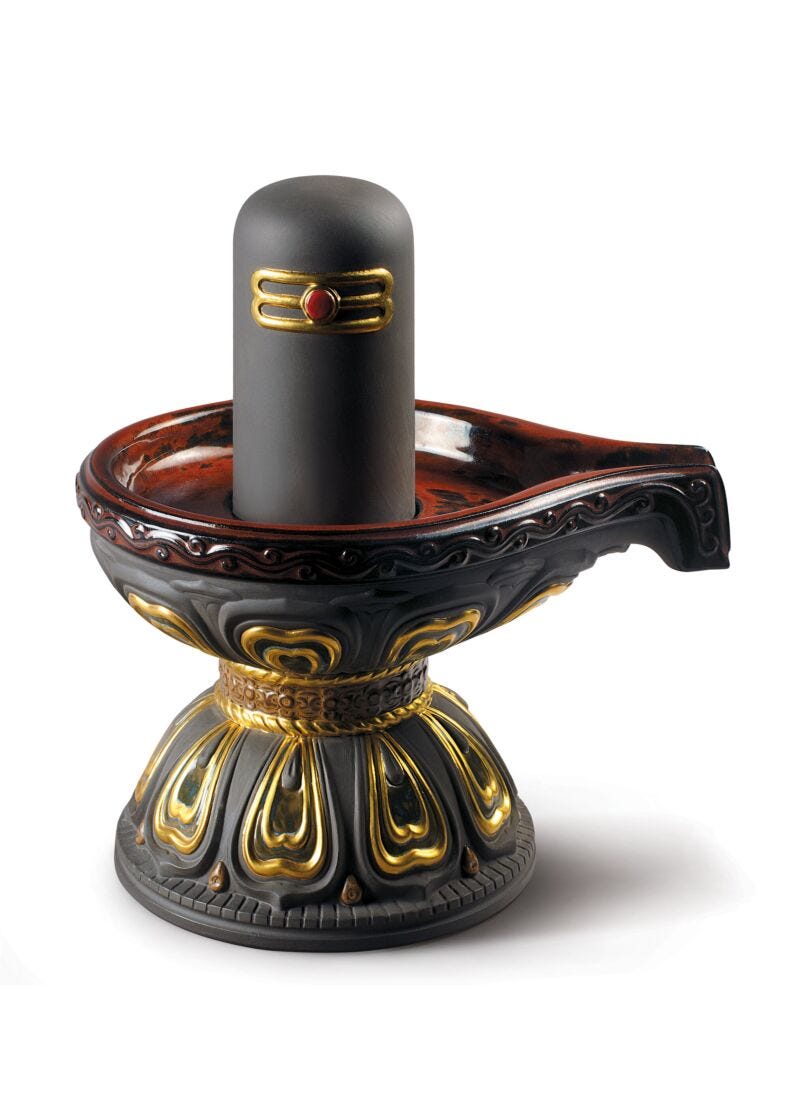This image features an intricately designed mortar and pestle of gray ceramic, accented with gold decorative elements. The base is a round, dark gray-brown bowl, which curves up and widens significantly to form an hourglass-like shape, with the top resembling a wider bowl. This upper section has a narrow edge, possibly for pouring, and prominent gold trim at various points, especially around the transition between the base and the upper bowl. The inside of the vessel appears to be lined with dark brown material. A tall, smooth gray cylinder stands in the center of the bowl, adorned with similar gold trim and a distinct red stone or raised carvings resembling back-to-back B's. The background is a plain white surface, highlighting the ornate details of the vessel. The overall design suggests influences possibly from Oriental or Egyptian aesthetics.